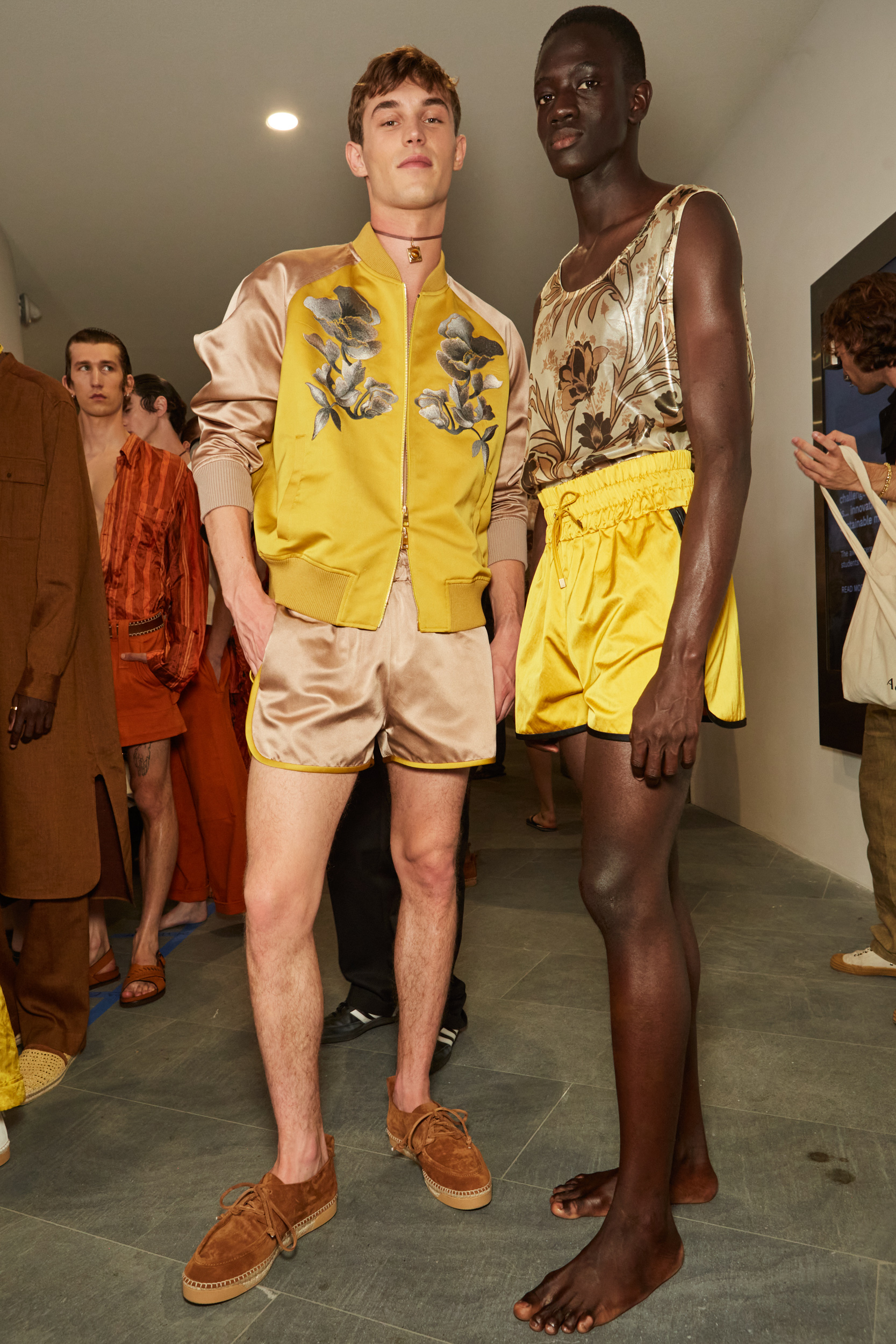In the image, taken indoors, possibly at a fashion show lineup, the focal point is two male models standing on a concrete floor. The scene is set against a beige wall with overhead lights visible on the ceiling. Positioned prominently at the forefront, the first model is a white male adorned in a striking ensemble: a gold jacket with floral designs on the chest, goldish shorts trimmed in yellow, brown shoes, and a choker. Beside him, the second model, a black male, wears a shiny floral tank top paired with yellow pull-tie shorts and is barefoot. To the left, a line of male models dressed in various outfits in shades of brown, orange, yellow, and beige are standing, possibly preparing for a show. One individual is seen standing against the wall, adding to the organized yet bustling atmosphere of a pre-runway setting.